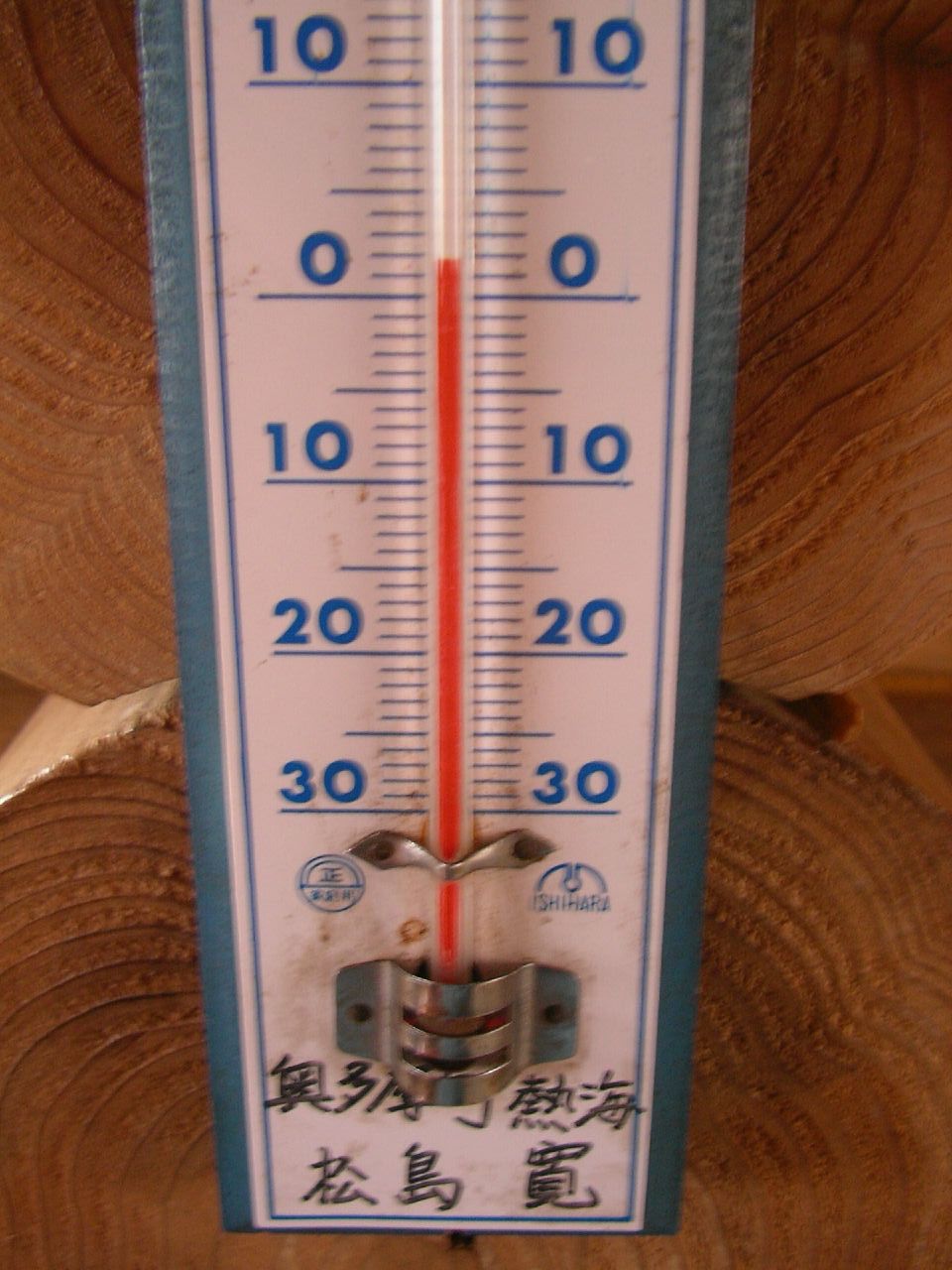The image depicts a partially visible thermometer mounted on a wooden surface. The thermometer features a blue border and is marked in blue numerals against a white background, suggestive of it measuring in Celsius. The visible scale ranges from -10°C at the top to 30°C at the bottom, with the red mercury indicating a temperature of approximately 2°C. The thermometer is affixed to the wooden base using two metal fasteners - a small one near the middle and a larger, thicker one at the very bottom for secure attachment. At the bottom of the thermometer, there is text written in what appears to be Japanese or another East Asian language, adding a distinctive touch to the device.